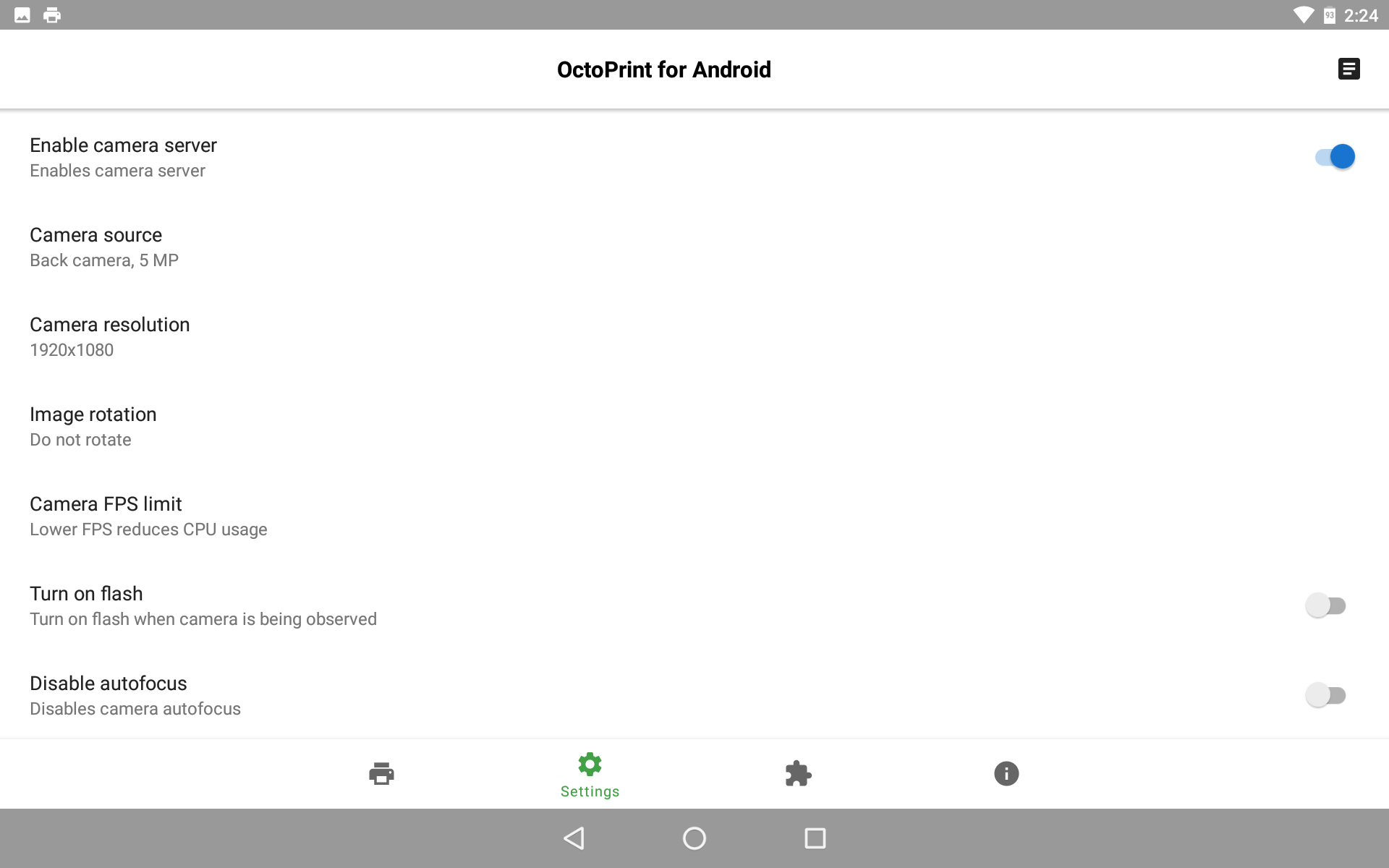Here is a detailed and cleaned-up caption for the described image:

---

The screenshot displays a user interface of an app, presumably "OctoPrint for Android." At the top, there's a thick gray bar, mirrored by a similarly thick gray bar at the bottom. On the right-hand side of the top bar, there is a "pick" icon and a printer icon, accompanied by the number "224." Directly below, it reads "OctoPrint for Android."

In the main section of the interface, a black box with horizontal lines is presented, under which lies a long gray line. Below this line, the text "Enable Camera Server" is shown, with an active toggle switch next to it.

Several camera settings are listed consecutively, starting with "Camera Source," followed by "Camera Resolution," "Image Rotation" with the value "Do not rotate," and "Camera FPS Limit." There is an explanatory note in gray that states, "Lower FPS reduces CPU usage."

Further down, the option "Turn on flash" is displayed in black text, with the note "Turn on flash when camera is being observed" in gray. Similarly, the setting "Disable Autofocus" is written in black, accompanied by the gray text "Disables camera autofocus." Each of these settings has its respective toggle switch.

Additionally, there is a thin gray line separating sections. Below this, the user interface shows a printer icon, a green settings icon, a puzzle piece icon, and a solid gray circle with a question mark in its center.

---

This caption provides a clearer, more structured description of the screenshot, highlighting the interface elements with respective colors and contextual details.